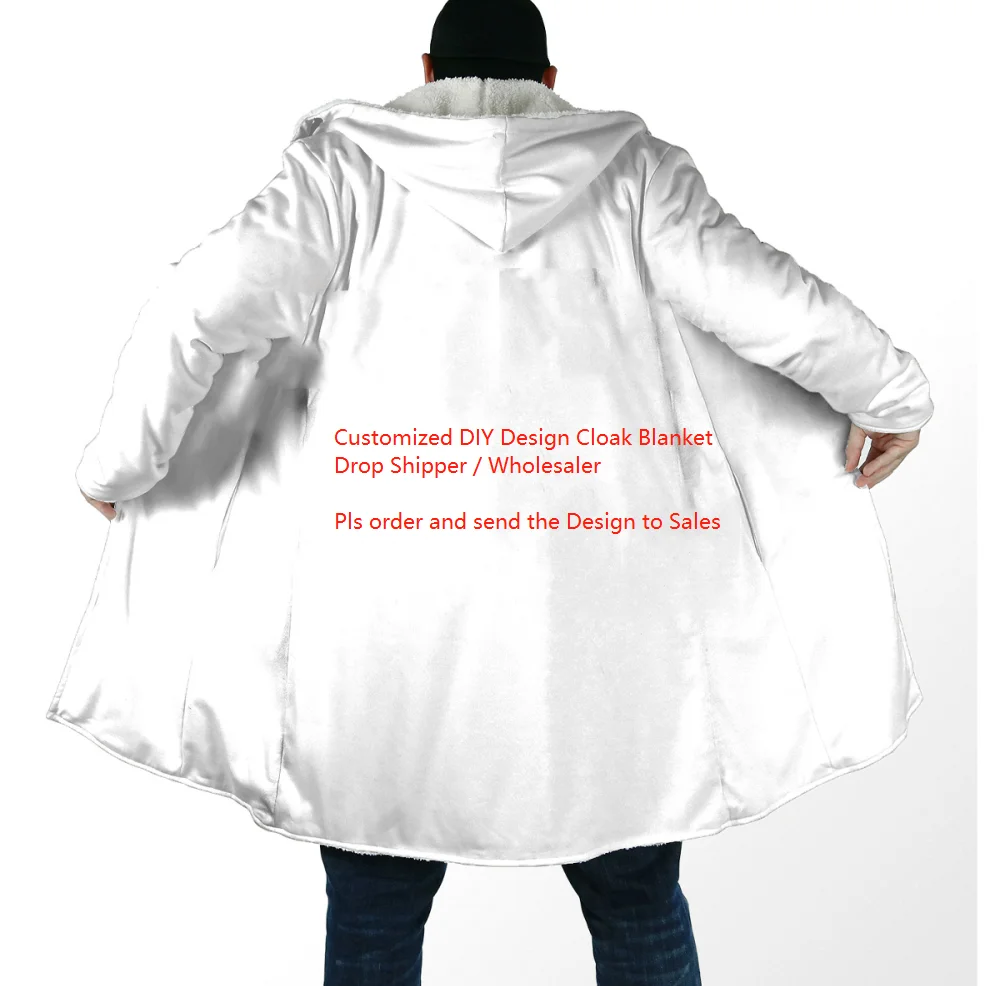In this image set against a largely white background with a hint of light gray in the bottom right corner, a man is depicted from the back. The photograph predominantly captures him from just above his knees and up, with the very top of his head cut off. He is wearing a thick, large cotton jacket with long sleeves and a white hood lined with fleece. The coat appears somewhat reflective and smooth on the surface, and the person is holding it open with both hands, revealing his fingers gripping the jacket's sides. A black beanie covers his head, exposing his ears underneath. The man is dressed in Levi dark blue jeans. Displayed prominently across the middle of the back of the coat is a red text that reads: "Customized DIY Design Cloak Blanket. Drop Shipper/Wholesaler. Please order and send the design to sale." This image seems to serve as an advertisement for a garment manufacturing factory.